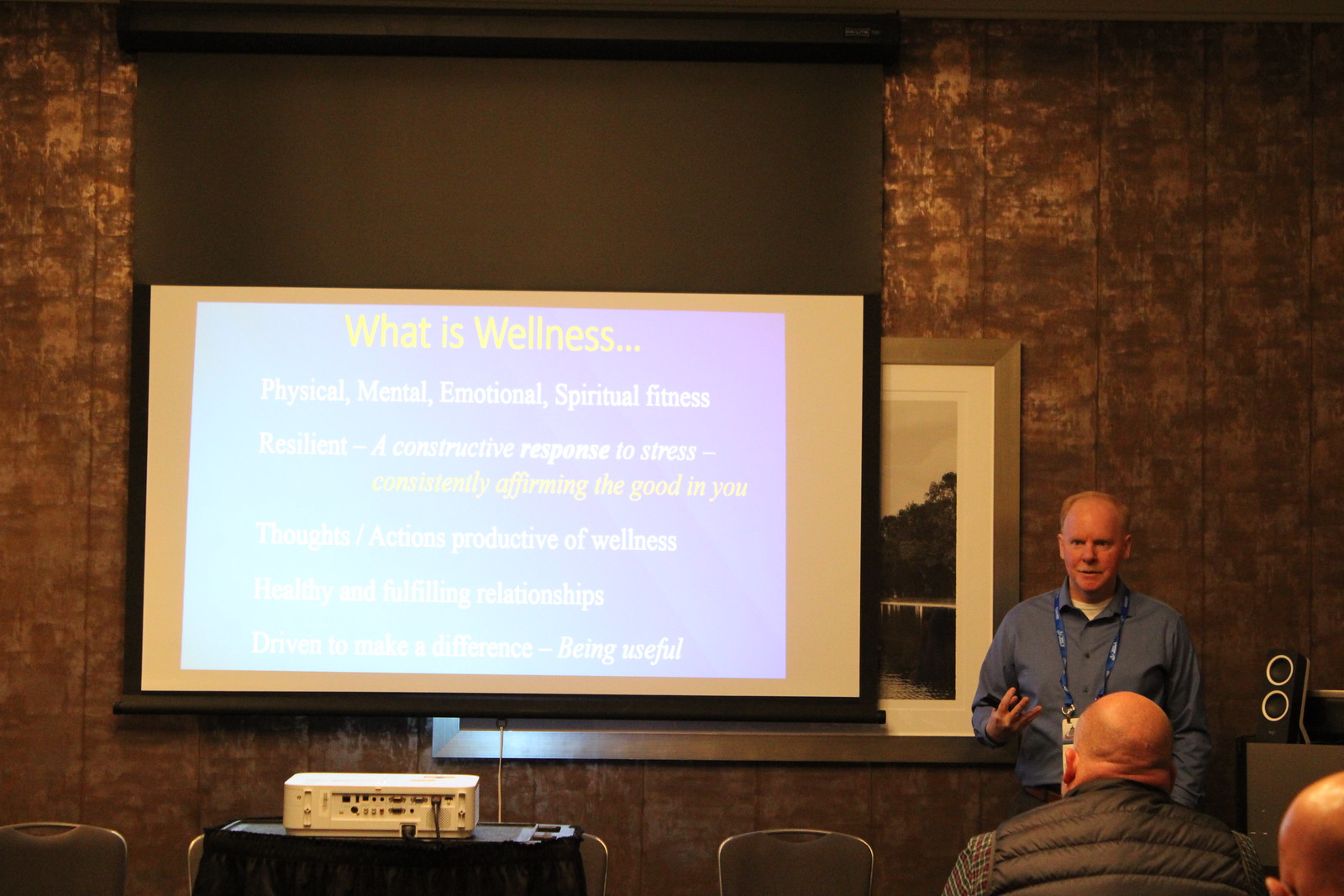The image depicts a motivational speaking event focused on the topic of wellness. At the center of the scene is a white projector screen displaying a slide with the headline "What is Wellness?" followed by sub-bullets including "Physical, Mental, Emotional, or Spiritual Fitness," "Realism, a Constructed Response to Stress," "Affirming the Good in You," "Product of Wellness," "Relationships," and "Be Useful." The text is primarily in yellow and white, set against a background that gradients from bright teal to fuchsia pink, creating a slight glare that makes some of the text difficult to read.

To the left of the screen stands a blonde man with thinning hair, dressed in a blue long-sleeve button-down shirt, black pants, and a blue lanyard with a name tag. He appears to have a white undershirt and a faint hint of facial hair above his lip. In front of the projection screen is a black table holding a white, square-shaped projector that resembles a printer.

The audience is seated to the right side of the image, with specific individuals wearing a black puffer jacket and flannel, and another man with a bald head partially visible. The room features a brown rustic wood wall adorned with a large, partially obscured landscape photo. Additionally, there is a speaker placed on a table or shelf in the right background. The atmosphere is one of focused attention, as participants listen to the presentation on wellness.